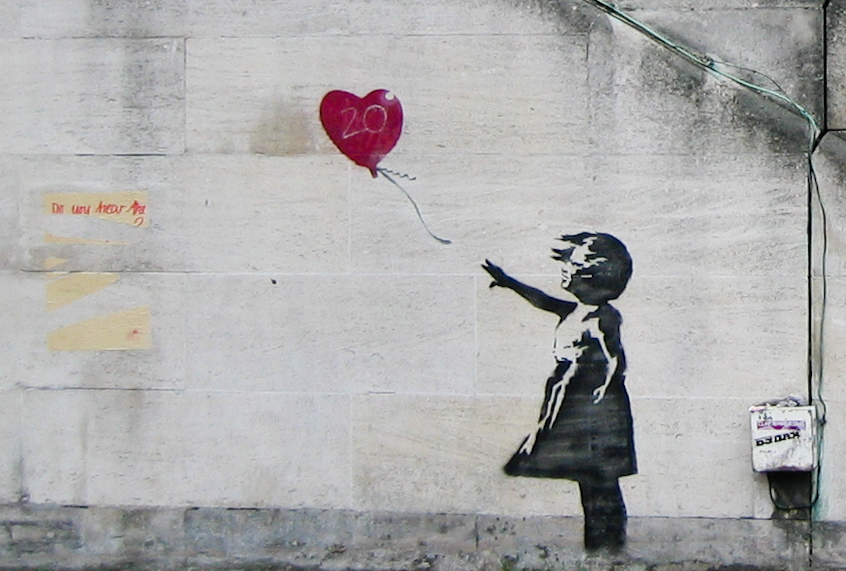This detailed mural, painted on a somewhat dirty white brick wall in an urban setting, features a striking black-and-white image of a young girl. Her right arm is outstretched, previously holding onto a red, heart-shaped balloon that has the number "20" written on it in white. The balloon is depicted being carried away by the wind to the left of the image. The wind also causes the girl's hair to blow across her face and her dress to billow out in front of her. There are signs of the mural being located in a bustling city environment, such as a torn, old poster and a power or telephone box situated on the right side. This piece of street art stands out not only because of its emotional depiction and the lone splash of color from the red balloon, but also due to the textured and weathered condition of the wall, adding to its urban charm.